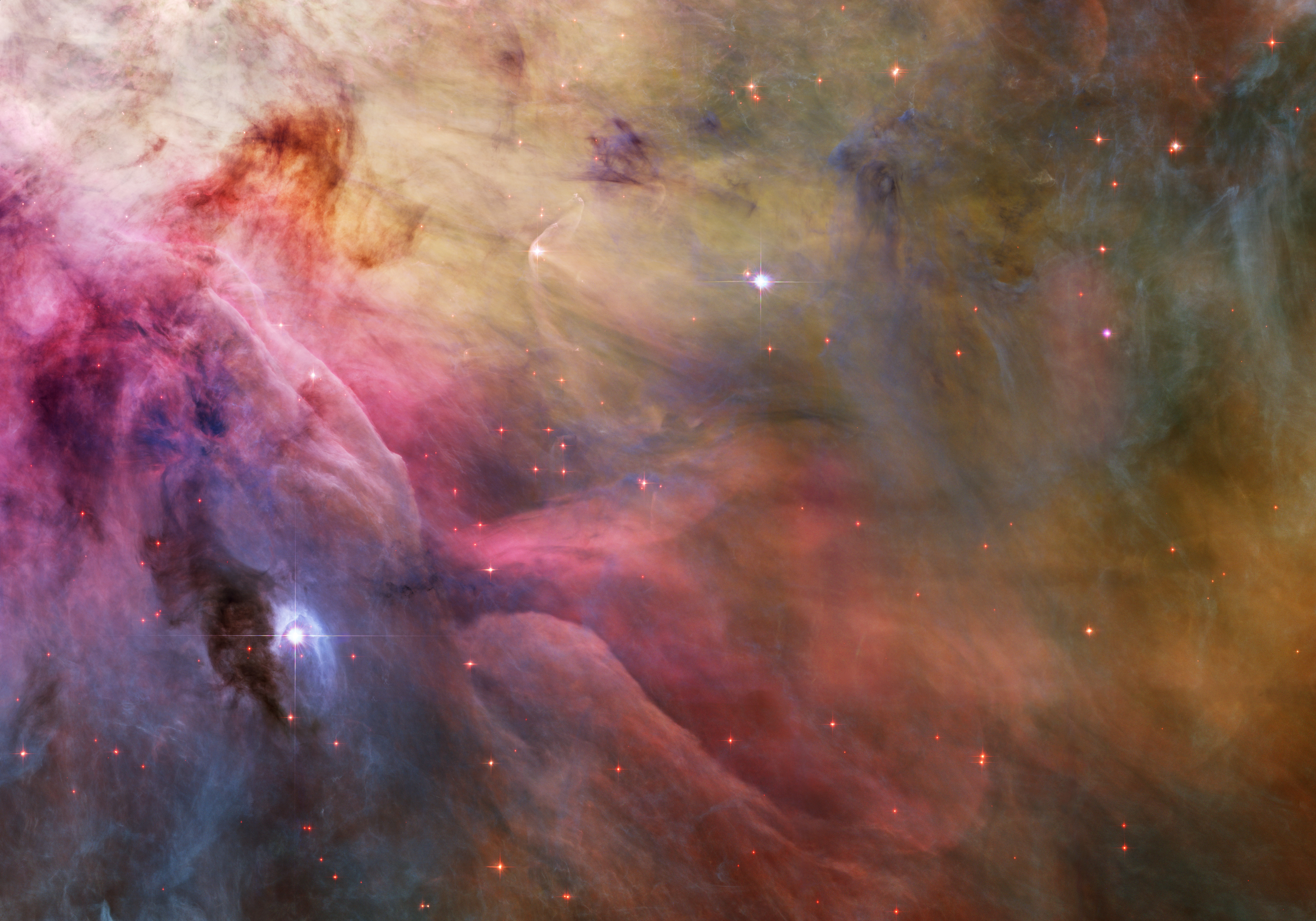The image presents a mystical, smoke-like appearance with an ethereal quality, reminiscent of a nebula in outer space. Swirling clouds of vibrant colors—ranging from blues on the lower left, transitioning through pinks and purples in the middle, and culminating in darker hues with light greens and browns towards the right—create a marbled effect. Bright spots of white light punctuate the scenery, with one prominent in the lower left and another near the middle top. Specks of gold and pink light are scattered throughout the image, enhancing its celestial ambiance. The interplay of colors and lights, along with the absence of any writing or symbols, lends the scene a dreamy, mysterious allure akin to cosmic phenomena.